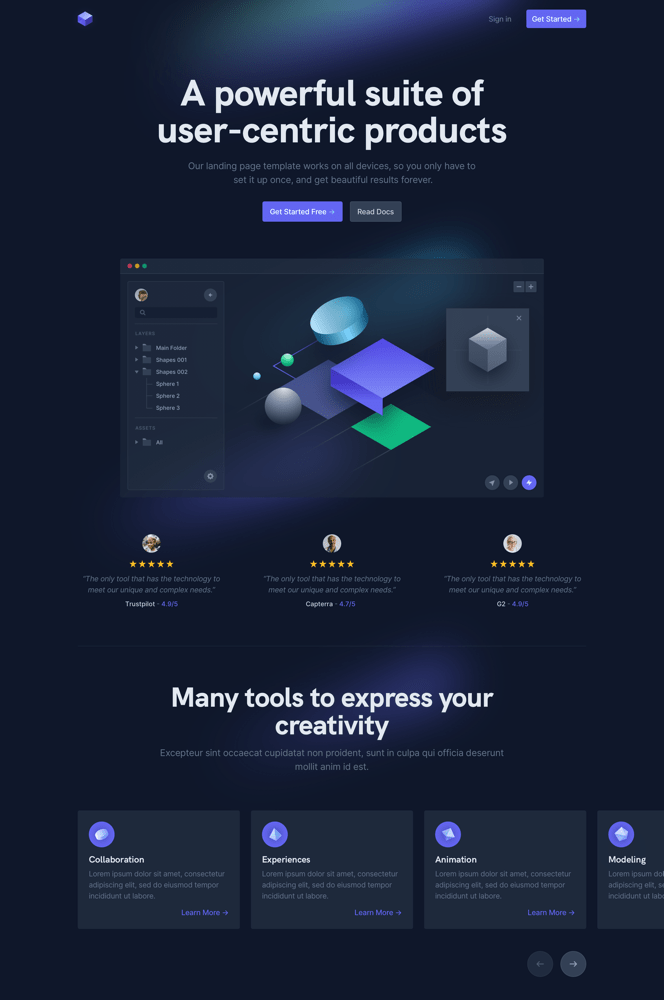The image displays a sophisticated and visually striking web page, characterized by a dominant midnight blue color scheme. The top right corner features a light blue "Get Started" button, while to its left, the "Sign In" text is somewhat difficult to read. On the far left, there's a small, blue geometric cube icon.

Central to the page, in a large white font, is the statement: "Powerful Suite of User-Centric Products". Below this is a description in smaller text: "Our landing page template works on all devices, so you only have to set up once and get beautiful results forever."

Below this text, the web page offers two prominent buttons: a blue "Get Started Free" button and a black "Read Docs" button. Beneath these buttons, a screenshot of an Apple MacBook is displayed, showcasing a multi-layered geometric shape. This shape includes a flat top layer with a side piece resembling a piece of paper, a floating halved cylinder, and key elements like planets, green spheres, and gray squares.

Additionally, to the left of the imagery, there are labeled file folders for layers: "Shapes" with subfolders "0012, 01, 02, 01, 02, and 03". Testimonial sections from "Trustpilot", "Capterra", and "G2" are also visible, featuring user reviews.

Further down, a large font text proclaims: "Many tools to unleash your creativity", accompanied by buttons labeled "Collaboration", "Experiences", "Animation", and "Modeling". Each box includes a clickable link to learn more. At the bottom of the page, navigation arrows are present with the left arrow grayed out and the right arrow active, allowing users to advance forward.